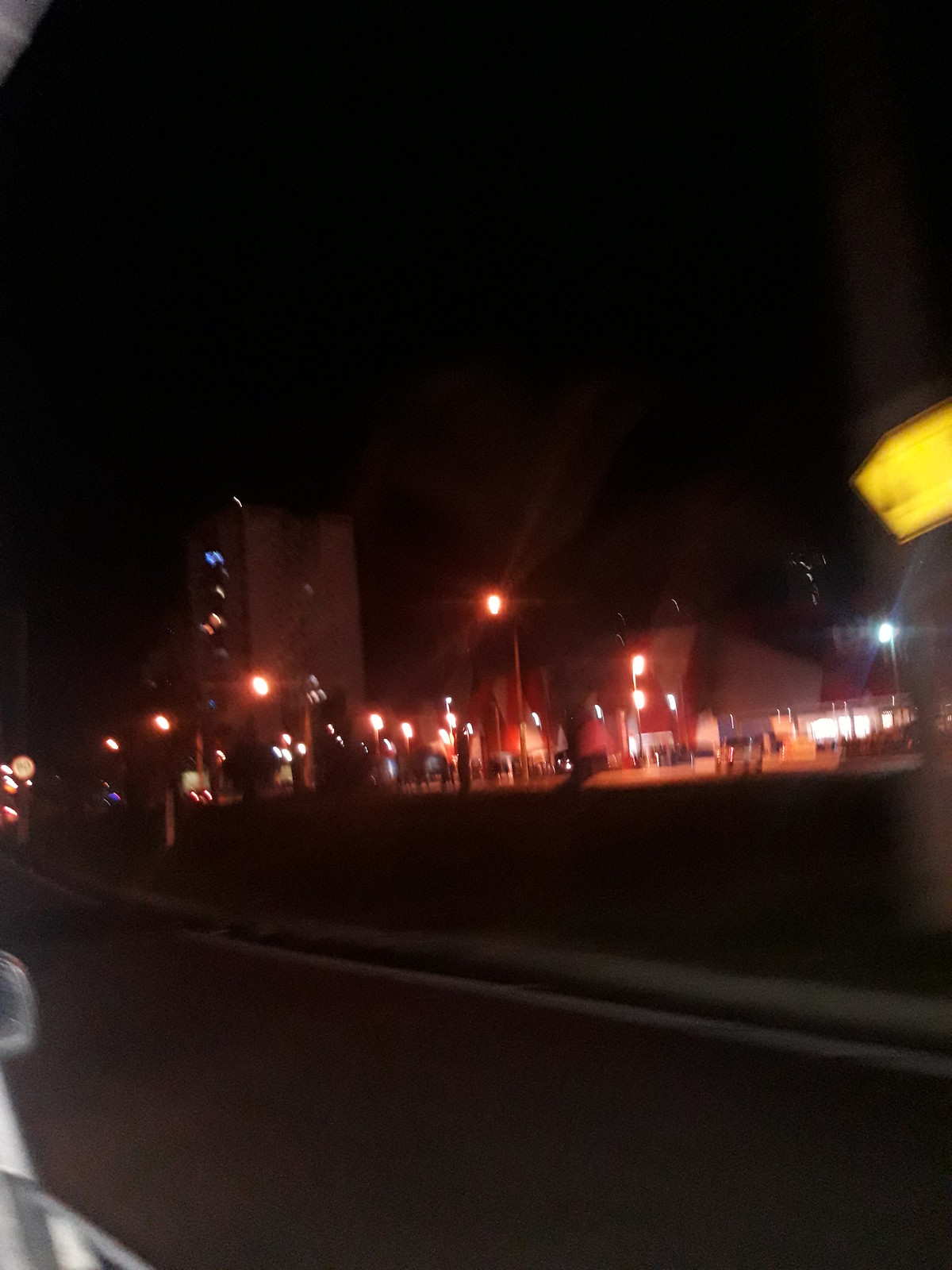The image depicts a nighttime scene of an urban shopping center. In the foreground, there is a large parking lot filled with numerous parked cars and illuminated by multiple tall streetlights emitting a bright orange light. Additionally, there are smaller streetlights of about half the height, also casting the same orange glow. Stretching across the horizon, a series of buildings with gray roofs and red sections have their entrances well-lit, providing a warm contrast to the dark surroundings. On the left side of the image, a tall building's windows are aglow with orange and blue lights, highlighting its height in comparison to the smaller buildings on the right side. To the right of the scene, the edge of a brightly lit building is visible. A small yellow rectangle can be seen in the upper right area of the photo, while a dark, black road with a white line runs alongside the parking lot. The entire scene is framed by a black, starless sky and a field of grass in the foreground, further emphasizing the urban night setting.